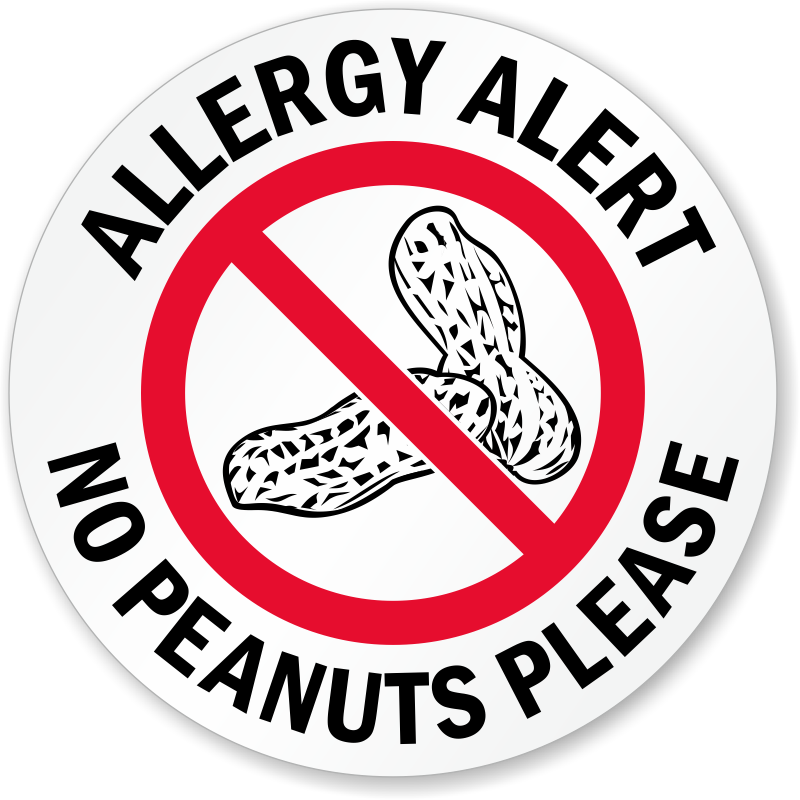The image is a square black and white illustration with spot color, depicting a round white sticker. Around the top rim of the sticker, in all caps black text, it reads: "ALLERGY ALERT, ALLERGY ALERT." The bottom rim features the phrase "NO PEANUTS PLEASE" in black text. The center of the sticker showcases a red circle with a diagonal slash running from the top left to the bottom right, symbolizing prohibition. Underneath the red circle, there is a detailed black and white illustration of two peanuts in their husks. One peanut is oriented slightly upwards to the left, while the other lies almost horizontally pointing towards the lower left. The background of the illustration is white, giving the effect that the sticker is floating. The combined elements clearly signify that peanuts are not allowed, highlighting an allergy alert.